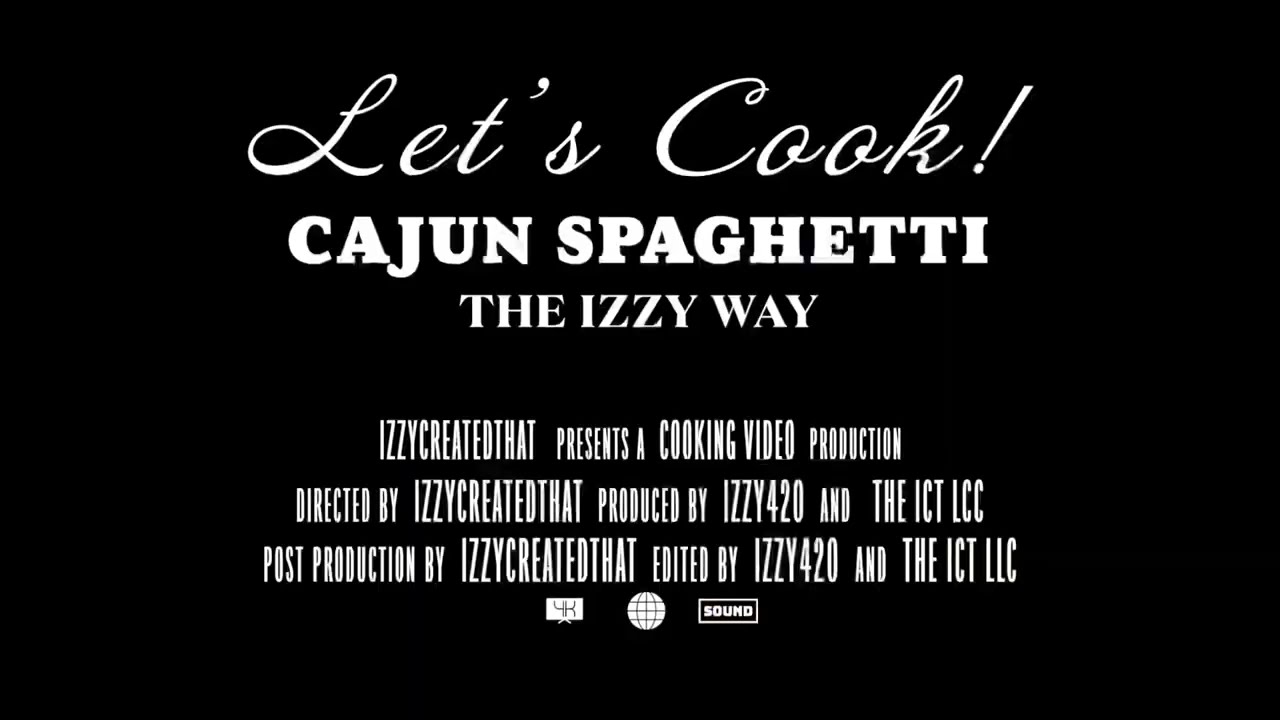The image showcases an advertisement styled as a vintage movie title card with a solid black background and white text. At the top, in cursive, it reads "Let's Cook!" followed by "Cajun Spaghetti the Easy Way" in normal, bolded text. Below this, it lists the creators and contributors in a format resembling movie credits: "Izzy Created That presents a cooking video production directed by Izzy Created That, produced by Izzy420 and The ICT LLC, post-production by Izzy Created That, edited by Izzy420 and The ICT LLC." At the bottom, there are three icons: a globe, a white square labeled "Sound," and a white box with "4K" indicating high-definition video quality.